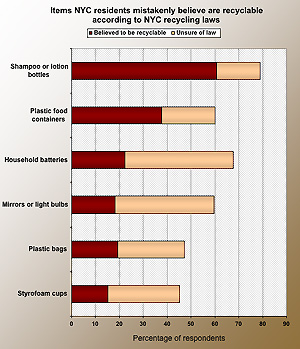The image is a gradient background chart transitioning from white at the top left to a light brown at the bottom right, illustrating items New York City residents mistakenly believe are recyclable according to NYC recycling laws. The chart features a mixture of red and cream-colored bars, with red indicating items believed to be recyclable and cream showing uncertainty regarding the laws. At the top, bold black text reads: "Items NYC Residents Mistakenly Believe Are Recyclable According to NYC Recycling Laws." The chart starts with shampoo or lotion bottles, showing about 65% of respondents believing these items are recyclable. Following these are plastic food containers at around 30%, household batteries at 20%, plastic bags at roughly 16%, and Styrofoam cups just below 12%. A Venn diagram or bar chart format is used to represent this data, with the graph’s x-axis indicating the type of items and the y-axis showing the percentage of respondents, ranging from 0 to 99%.